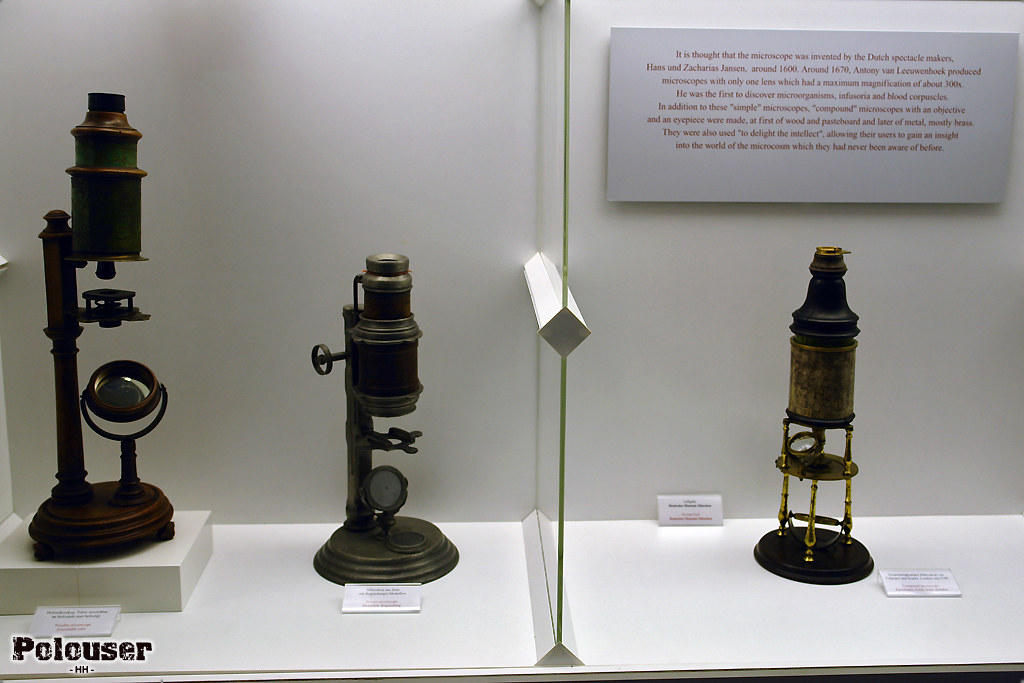This photograph, taken in what appears to be a museum, showcases a meticulously illuminated display case divided into two sections by a central glass pane. The backdrop and floor of the case are white, creating a stark contrast against the antique objects inside, which seem to be early microscopes. 

On the left side of the display are two microscopes characterized by their intricate metal structures. Both have a small metal platform, topped with two vertical stalks. The foremost stalk features a small magnifying lens, while the taller one supports the cylindrical tube through which users would peer. The base of these microscopes holds a tiny mirror, essential for redirecting light onto specimens.

The right side contains a single microscope, distinct in its construction with a more unified form. This piece has a gold metal structure forming a rounded top and cylindrical body. It appears less segmented compared to its counterparts and has a black base, further emphasizing its antique nature.

In the lower left corner of the display, there's a watermark that reads "POLOUSER" followed by what seems to be the characters "HH." Beneath each microscope lies a white label, though the text is too small to decipher.

Mounted above the right-hand section is a gray sign with red text. While partly legible, it discusses the invention of the microscope by Dutch spectacle makers Hans and Zacharias Janssen around 1600, and notes the advancements in microscope design around 1670, which included lenses with a magnification of up to 300x. The text also highlights the evolution from simple to compound microscopes, which were initially made from wool and parchment board and later from metal, mostly brass, fundamentally expanding users' understanding of the microscopic world.